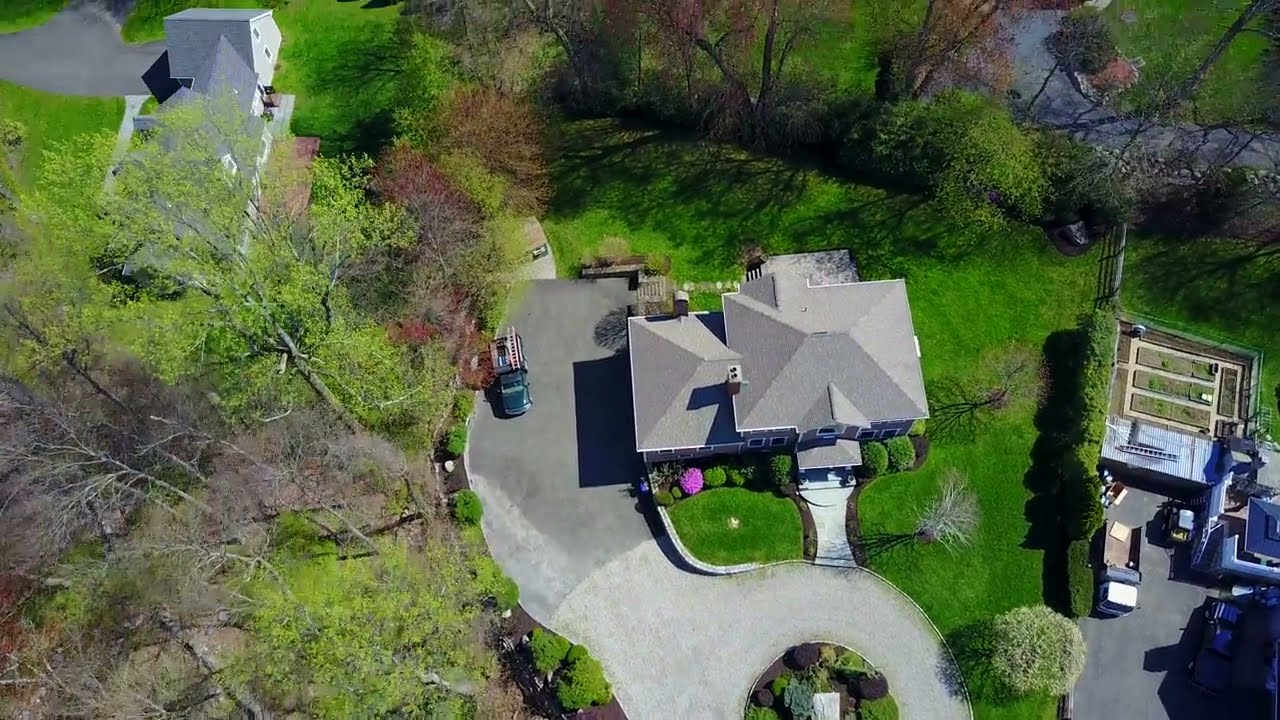This aerial photograph captures a two-story house with a gray shingled roof, featuring a chimney in the bottom left corner. The home, surrounded by well-maintained, lush green grass, boasts a neatly trimmed lawn with various shrubs adjacent to the house, including one that's distinctly bright pink. The front entrance is highlighted by a covered walkway made of gray concrete leading to a circular driveway, which extends to the left side of the house, providing ample parking space.

In the driveway, a green pickup truck is visible, loaded with some slanted objects in its bed. To the left of the truck lies a dense forest, populated with both vibrant green and bare brown trees. The backyard reveals a large grassy area leading to another tree line, predominantly filled with green leaves and enclosing an upper-right-corner roadway. Between the house and an adjacent building situated in the bottom left corner, separated by a barrier and fencing with shrubs, there's an industrial building with a box truck on a small asphalt path.

The clear, sunny day allows for a crisp view, emphasizing the greenery and detailed elements, such as the box truck and another roundabout driveway leading to additional homes at the top edge of the image. No people are visible in this serene and detailed overview of the property's landscape and surrounding area.